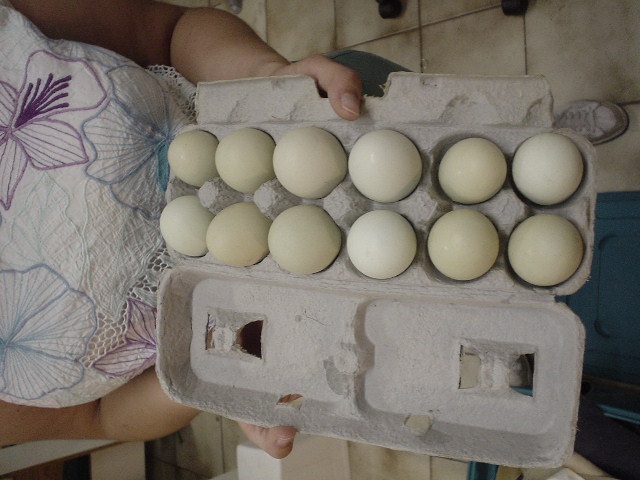The image features a young girl, dressed in a white dress adorned with embroidered flowers in shades of blue and purple, standing on a beige tiled floor. She holds an open gray paper egg carton in front of her with both hands, her thumbs visible on top. The carton contains 12 eggs of varying sizes and colors, suggesting they are fresh duck eggs rather than store-bought. The eggs range in color from pure white to shades of light blue, grayish-yellow, and even some with bluish or orangish hints. The girl is wearing white sneakers, and the photograph, taken with an actual camera, is turned slightly sideways.